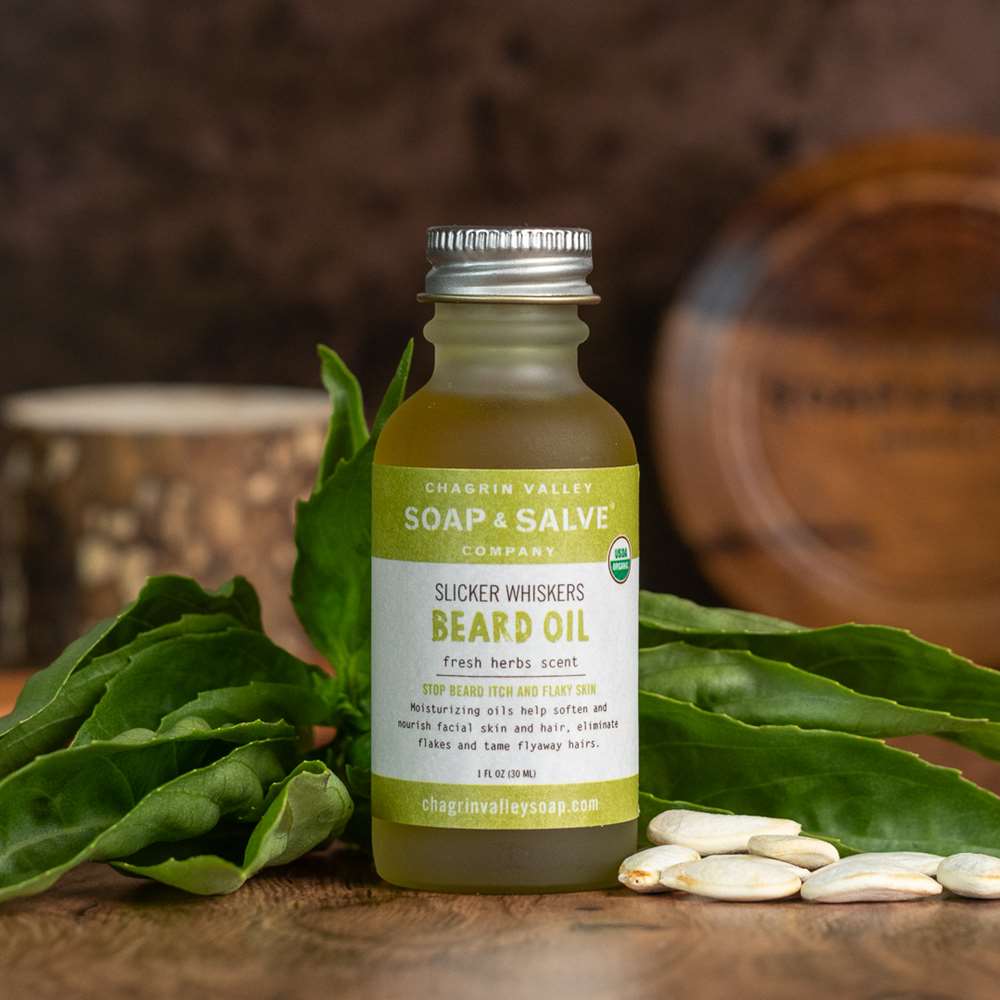The image showcases a close-up, indoor photograph of a bottle of Chagrin Valley Soap and Salve Company Slicker Whiskers Beard Oil. The bottle, approximately five to six inches tall, is plastic with a silver screw-on cap and contains an amber-colored liquid. The label features green sections at the top and bottom, with a white center, and reads: "Chagrin Valley Soap and Salve Company, Slicker Whiskers Beard Oil, Fresh Herb Scent. Stop beard itch and flaky skin. Moisturizing oils help soften and nourish facial skin and hair. Eliminate flakes and tame flyaway hairs." The label also indicates the product size as one fluid ounce (30 milliliters) and provides the website, chagrinvalleysoap.com.

The bottle is displayed on a wooden table, surrounded by green leaves and pods, along with some white seeds positioned to the right. In the background, there is a blurred image of a wooden plate standing up and a brown pottery cup with beige circles. The overall setting is earthy and complements the natural essence of the beard oil product.